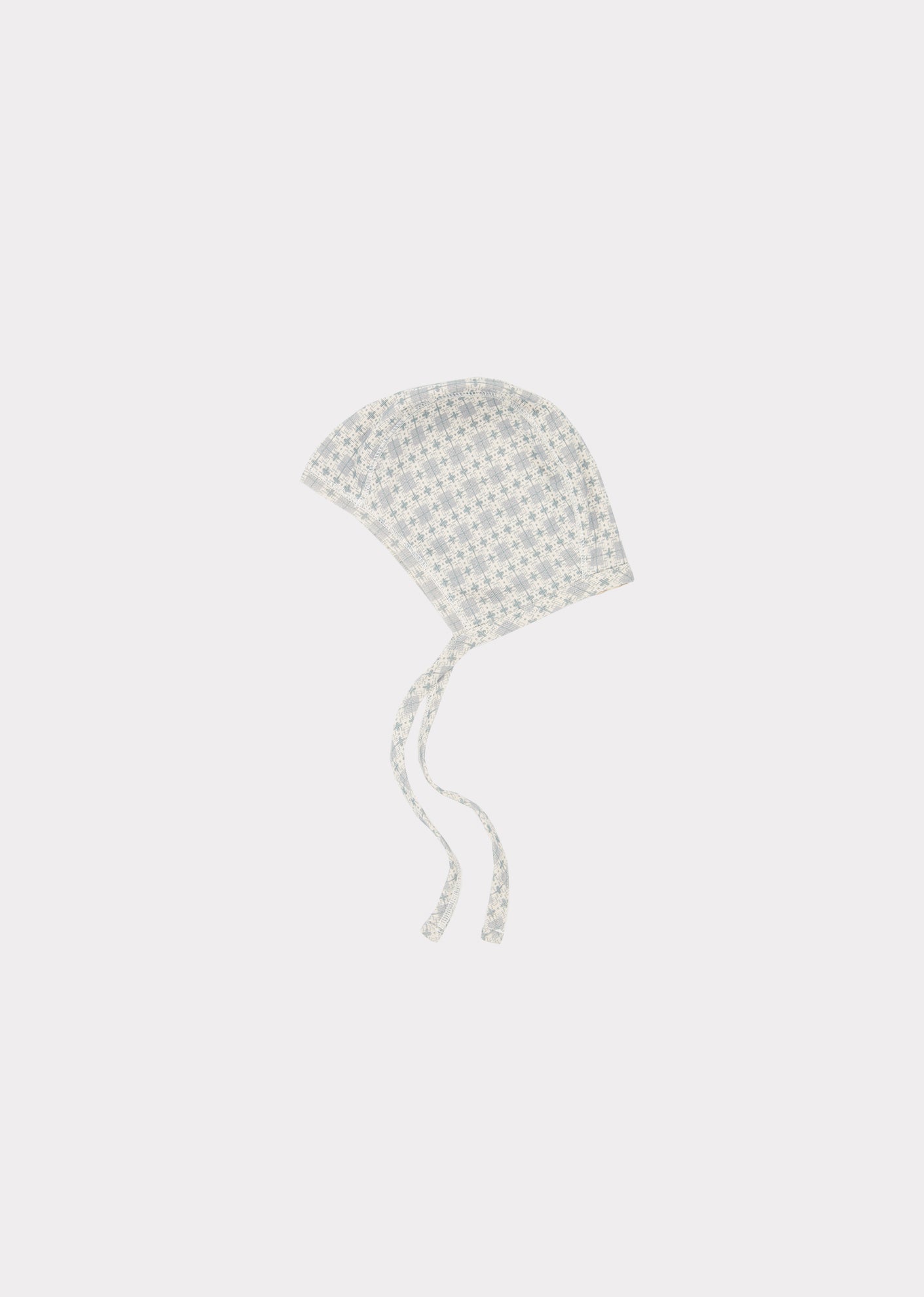The image depicts a small, possibly vintage, bonnet suitable for a baby or toddler, specifically designed for a girl. The bonnet is woven from lightweight cotton and features long straps meant to be tied under the chin. It is adorned with a detailed all-over graphic pattern consisting of alternating purple squares and green stars or diamonds. The illustration is set against a minimalistic, light blue background, centered slightly above the midpoint of the image. The overall design suggests it could be handmade, lending a nostalgic charm to the accessory.